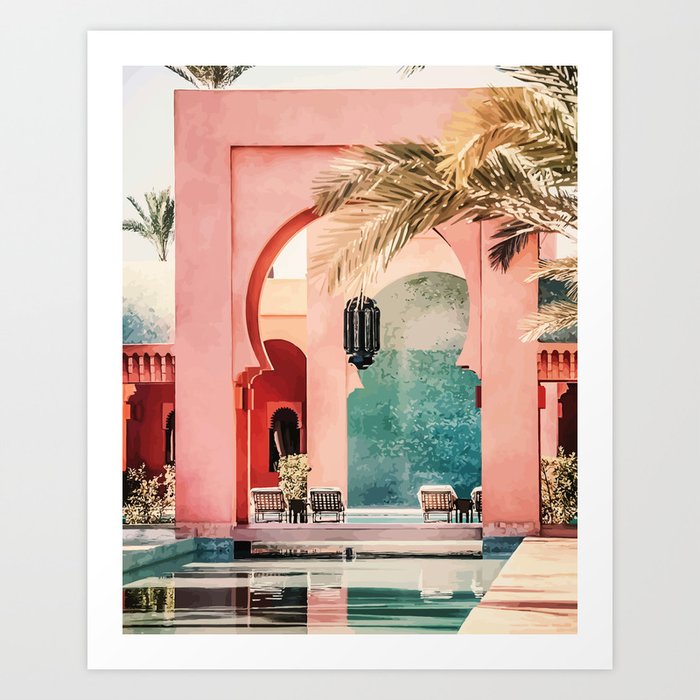The image depicts an artistic and vividly detailed watercolor painting of a serene, tropical poolside scene that gives off relaxed Istanbul vibes. At the center of the composition is a freestanding, grand archway painted in shades of purple and pink, positioned at the end of a glistening, clear, water reflection pool. The arch supports a large, hanging lantern and is flanked by multiple lounge chairs. The foreground and background feature lush green palm trees, set against a soft, light-colored sky that further contributes to the scene's tranquility. A series of smaller plants and bushes dot the area around the pool, enhancing the tropical atmosphere. In the background, a Mexican-style, coral-pink building with distinctive windows and a wall adds architectural interest to the composition. The scene combines shades of muted green, blue, tan, and coral, creating a harmonious and calming visual experience. The overall effect of the painting is both exotic and inviting, making it reminiscent of a refined postcard image.